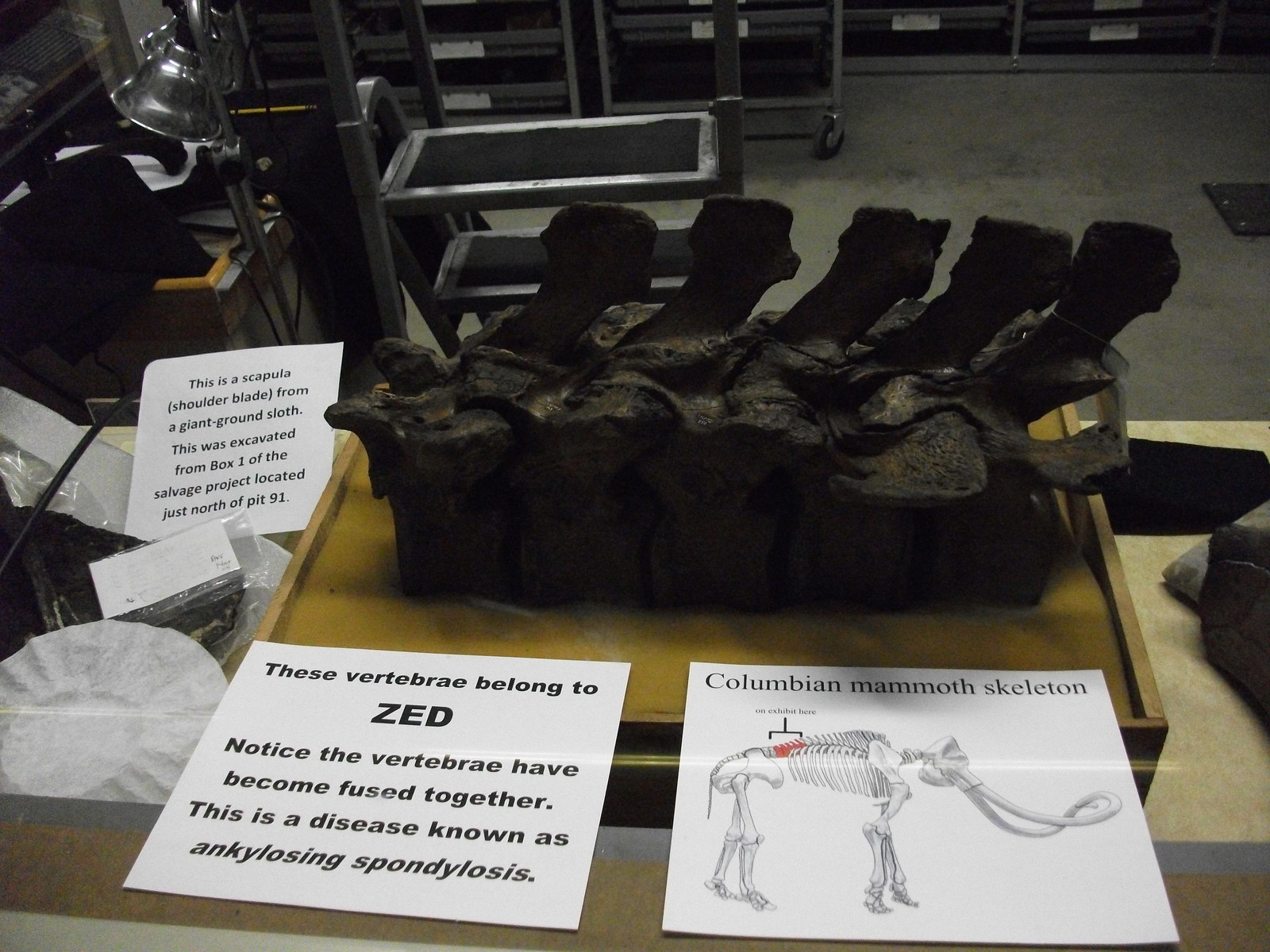The photo showcases an aged and blackened vertebra, possibly from a mammoth, clearly displaying signs of fusion consistent with ankylosing spondylosis. Three pieces of paper accompany the vertebra: one on the lower left identifies the specimen with the note, "these vertebrae belong to Z," and highlights the disease causing the fusion. To the right, a printed sheet titled "Columbian Mammoth Skeleton" includes a black-and-white skeleton diagram with a red-marked section indicating where the vertebra would fit. The leftmost paper describes a scapula from a giant ground sloth, specifying its excavation from box one of a salvage project near pit 91. The background features a concrete floor and various storage units, indicating an archival or exhibition preparation area.